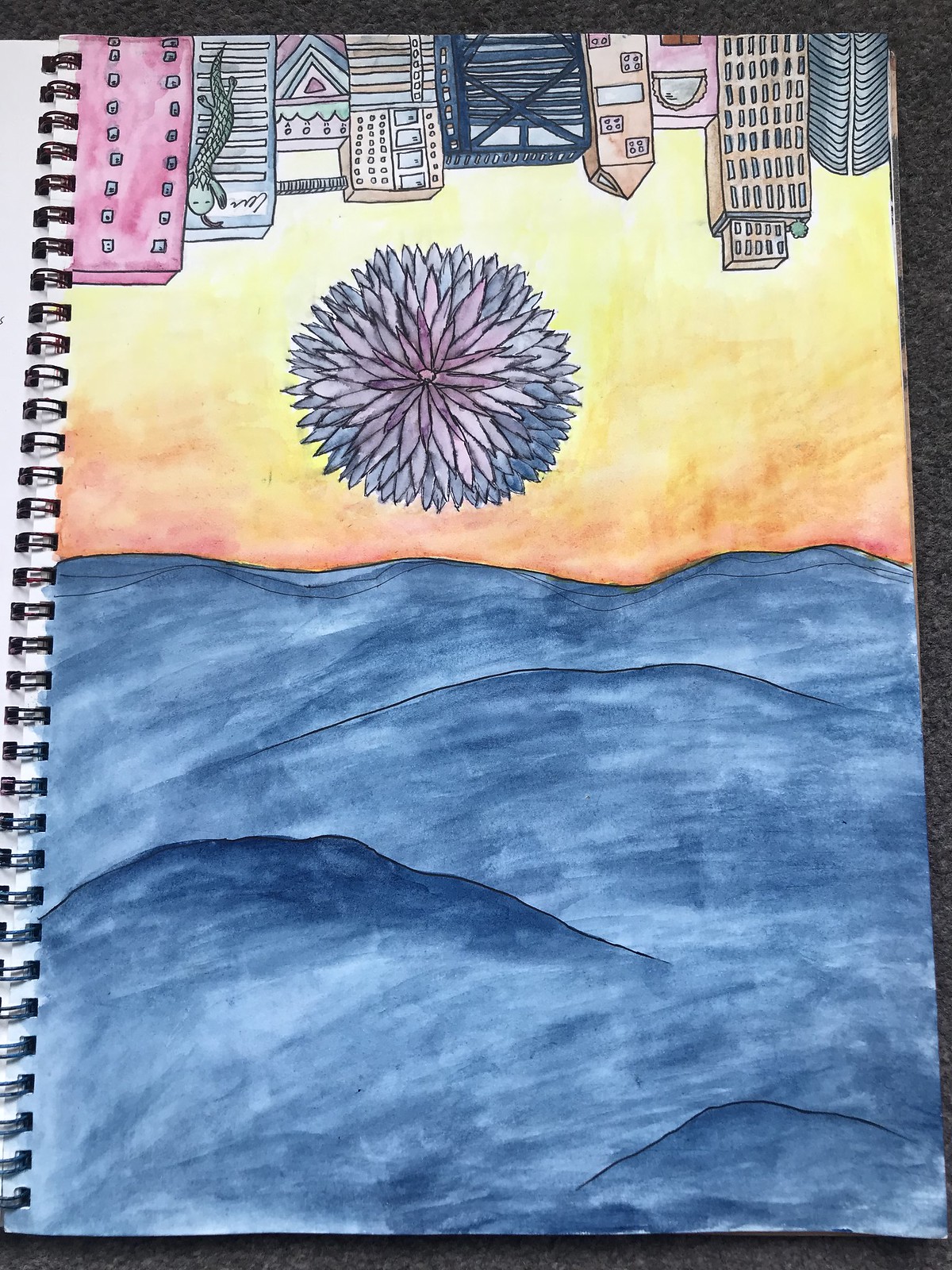This detailed color illustration, seemingly executed in watercolor paint on a spiral-bound sketch notebook, captures a surreal coastal scene with vivid and contrasting elements. At the bottom of the image, dark hills or mountains, almost black in color, anchor the composition, creating a stark contrast against a beautifully painted horizon that transitions from a deep orange to a soft yellow, evoking the hues of a setting sun. 

In the center of the image, a striking flower or sea anemone with light pinkish-purple petals serves as the focal point. This floral element exhibits a delicate gradient, fading to darker shades at its edges, drawing the viewer's eye.

Above the flower, blue waves, outlined in black ink and possibly filled in with blue marker, add to the coastal theme with their rhythmic patterns. At the top of the illustration, upside-down skyscrapers or tall buildings are depicted, creating an intriguing and disorienting perspective. This inversion effect suggests a dreamlike scenario where the sky meets the cityscape, blending reality with imaginative artistry. The overall composition conveys a vivid blend of natural and urban elements, seamlessly merged through vibrant watercolor techniques.